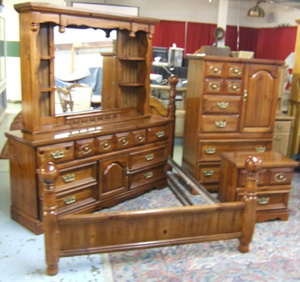The image is a detailed, color photograph in landscape orientation, showcasing a matching set of bedroom furniture in what appears to be a store environment. The set, crafted from dark brown wood, includes a spacious bed frame with circular posts, a large wooden armoire, a dresser, and a smaller side table. The armoire features a mix of cabinets, drawers, and shelves, with brass handles adorning its drawers. To its right, there is a tall chest that boasts a combination of large and small drawers, with an openable, arched-top drawer on the right side. In front of this chest sits a two-drawer nightstand. All these pieces rest atop a large rug featuring a white border and multiple blue, pink, and white lines. The background reveals a store setting, with the lower half of the wall covered by a red curtain and the upper half painted red. A white support pillar stands in the top left corner, with a light fixture featuring a gold lampshade in the top right corner, adding a touch of elegance to the scene.